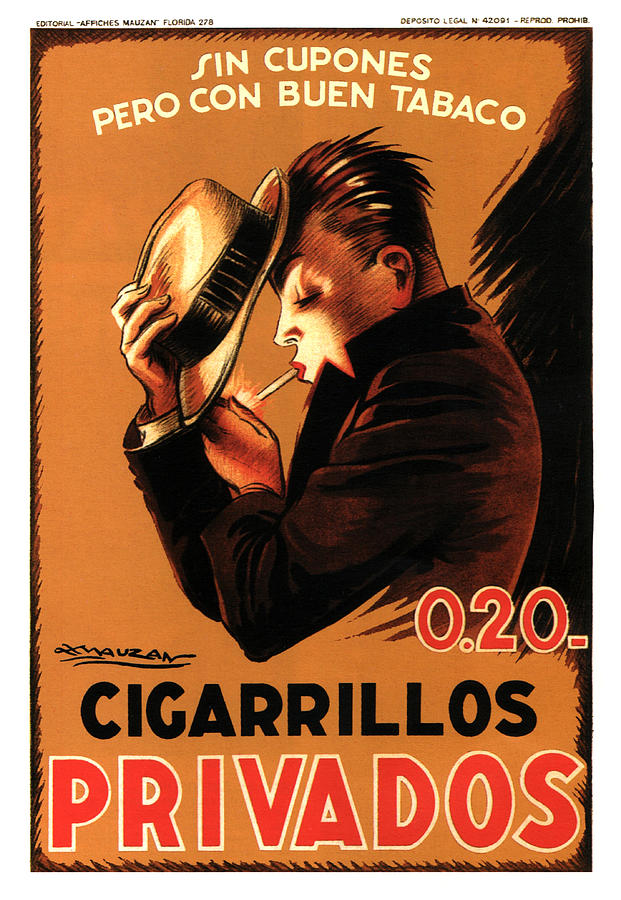This is a vintage advertisement poster, likely for cigarettes, featuring an illustration of a person with striking red lips lighting a cigarette. The poster has an orange background with a dark brown border that creates a shadow effect. The illustration shows the character facing left, with their head tilted down as they light the cigarette, using their right hand to hold a hat, which is yellow with a brown band, in front of their face. Above the illustration, there are two lines of white text reading, “Sin Coupones Pero Con Buen Tabaco.” Below the character, in black text, it says “Cigarillos” and beneath that in red text with a white outline, “Privatos.” The price “0.20” is displayed prominently in the bottom right corner. The poster includes an old-fashioned vibe, with additional text on the outer edges mentioning "Editorial-Mefiche's Mouson Florida 278" on the left and "Deposito Legal N 42091," with notes indicating it's a reproduced and prohibited item. The details and sketch-like quality emphasize its antiquated and stylized appearance.